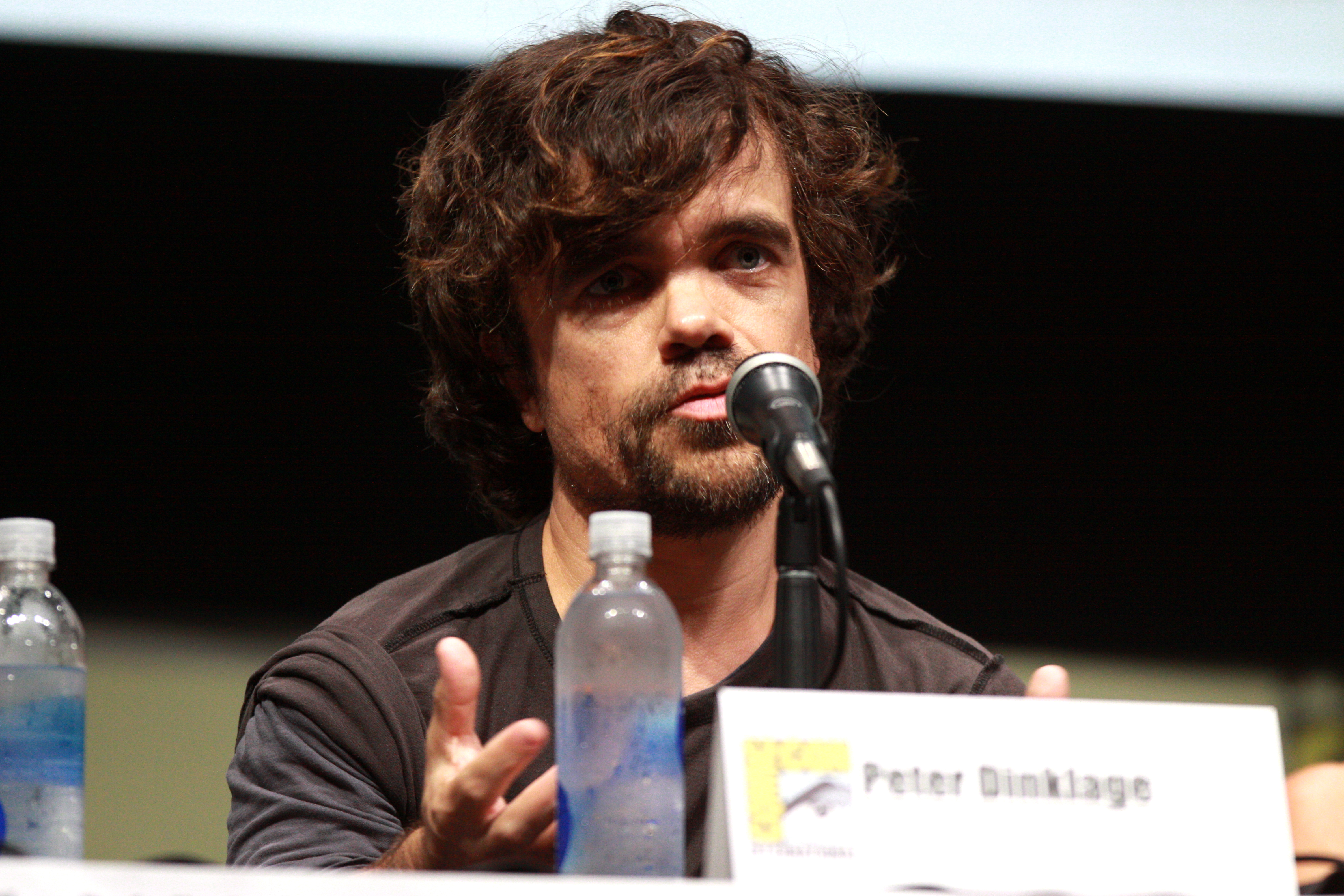The image captures a close-up of actor Peter Dinklage, known for his role in Game of Thrones, sitting at a convention panel, likely Comic-Con. Peter Dinklage, a dwarf with medium-length, wavy brown hair that falls into his forehead, is addressing the audience in front of a black and silver microphone. He is wearing a grey t-shirt and gesturing expressively with his hands, his right hand palm up and fingers extended. On the table in front of him are two bottles of cold water, both featuring white caps and blue labels, with one placed directly in front of him and another to his left. A white name card with blue lettering reading "Peter Dinklage" and a yellow Comic-Con symbol sits prominently on the table. The background features a gradient from dark black at the top to a lighter shade at the bottom, with a white ceiling visible above.